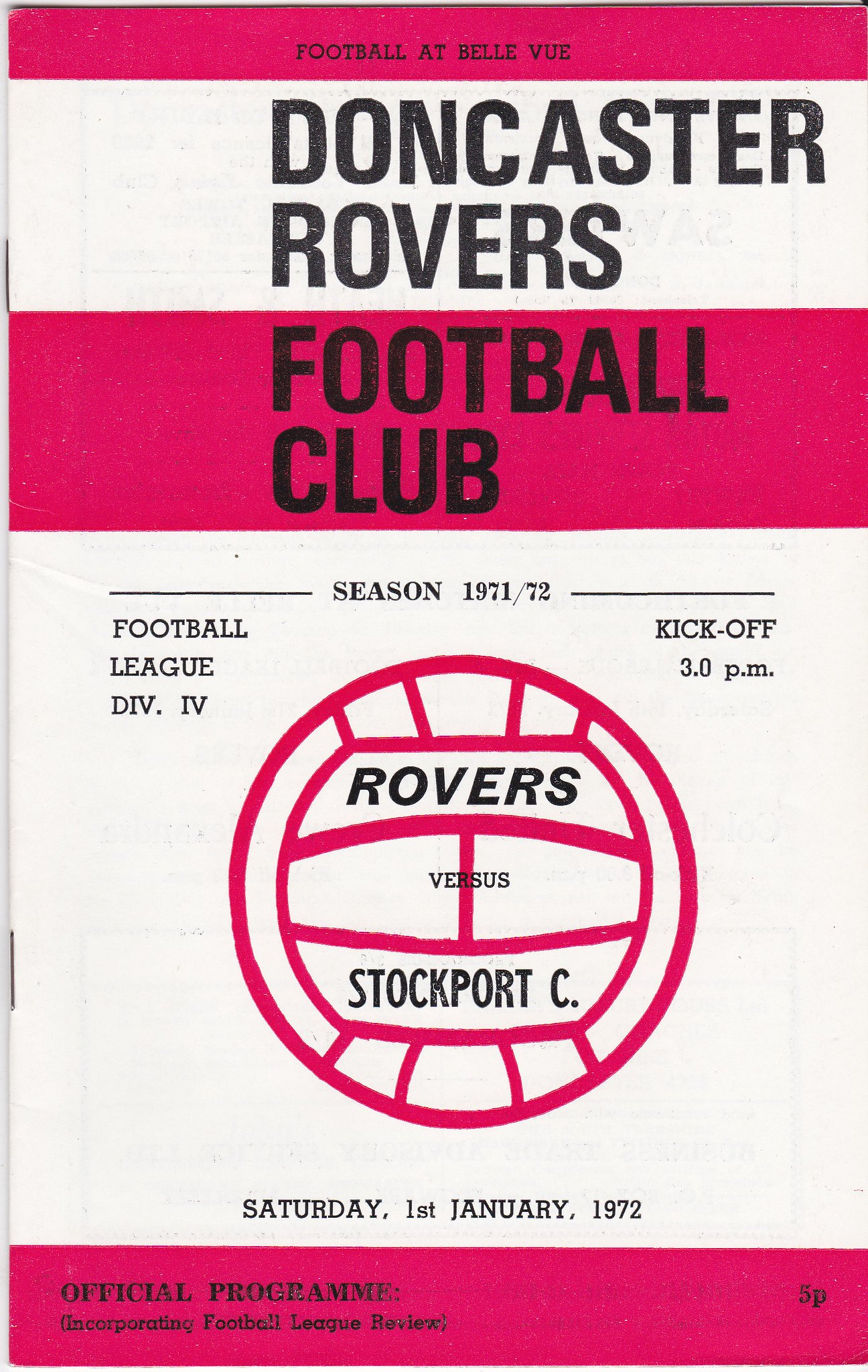This image is a scan of a vintage football match program cover for Doncaster Rovers. The design predominantly features red, white, and black colors. At the very top, a red bar spans the width of the cover with the text "Football at Bellevue" in bold black capitals. Directly below, a white bar with bold black letters displays "Doncaster Rovers." Following this, another red bar reads "Football Club" in black text. The main section of the cover features details about the game, starting with "Season 1971-72 Football League Division Four Kickoff 3pm" in black text over a white background. Central to this section is a red-outlined drawing of a soccer ball, inside of which "Rovers vs. Stockport C" is written in black text. Further details include the match date, "Saturday 1st January 1972," followed by another red bar stating "Official Program Incorporating Football League Review" in black text. In the bottom right corner, it indicates the price, "5P."